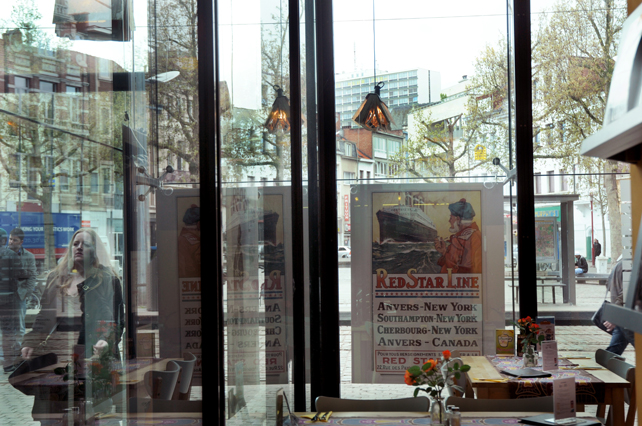This photograph captures the interior of a quaint, stylish café with high ceilings and large, floor-to-ceiling glass walls featuring black partitions. The foreground showcases a wooden table adorned with a floral runner, a small vase containing three red or orange flowers, and a matching wooden chair. Another similarly set table is visible in the corner. The windows display the reflection of a woman on the far left pane and are adorned with an intriguing vintage poster. The poster prominently features the text "Red Star Line" in bold red letters, accompanied by an illustration of a man, reminiscent of an old sea captain wearing a Scottish-style hat with a pom-pom, gazing at a large ocean liner. Beneath the illustration are the destinations listed: "Anvers, New York, Southampton, New York, Cherbourg, New York," and "Anvers, Canada." Ambient light filters through the café from a distinctive lighting fixture resembling an open book. Beyond the windows, the bustling cityscape unfolds, with people walking along the sidewalk and multi-story buildings framing the urban scene.